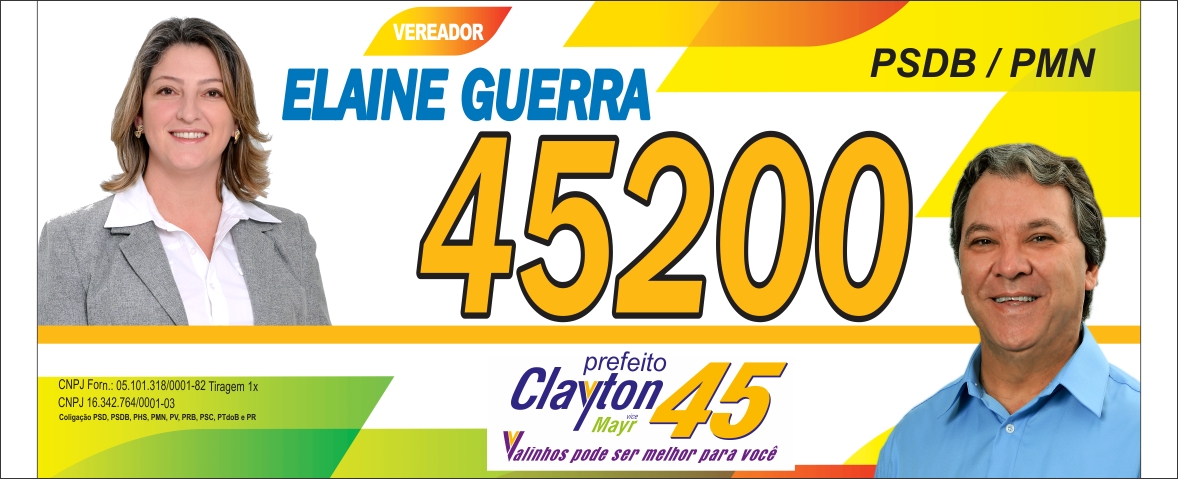The image appears to be a Spanish-language political advertisement featuring two individuals. On the left side, there is a professionally dressed woman with a gray blazer and a white dress shirt, identified as Elaine Guerrera. She has blond hair and is smiling. Next to her name in blue, there's a small orange banner that reads "Verador." Centered prominently below her name are large yellow numbers "45200" underlined by a yellow banner, suggesting some significant numerical detail.

On the right side of the image stands a man with grayish hair, a tanned complexion, and a blue dress shirt. He is also smiling. The ad features colorful designs with elements in green, yellow, and orange. To the right of the central text, there's a square yellow sign with a touch of lime green that displays the text "PSDB/PMN" in black letters. 

Finally, below the central numbers "45200," the text "Perfetto Clayton Mayor" appears in lime green, possibly indicating the man's name and the position he is running for. Additional colorful elements in purple and light green decorate the lower portion of the image, reinforcing the vibrant and eye-catching design intended to draw voter attention.